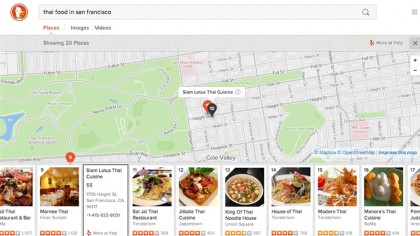This image is a detailed screenshot from a food search web page, likely related to Yelp. At the top, a gray search bar displays the query "Thai food in San Francisco." Next to the search bar, there is an icon depicting a duck in a red circle. Below the search bar, there are three tabs labeled "Places," "Images," and "Videos," with the "Places" tab currently selected.

The main section of the image features a map centered on San Francisco, pinpointing a restaurant named Siam Lotus Thai Cuisine, which is located just east of Golden Gate Park. In the upper right corner of the map, there is a link labeled "More on Yelp" accompanied by the Yelp logo.

On the left side of the image, a panel indicates that 20 places are being shown. This panel includes a list of numbered options, displaying entries 8 through 17. Siam Lotus Thai Cuisine is listed as number 10. Each listing provides the restaurant's name, photos of dishes, and star ratings.